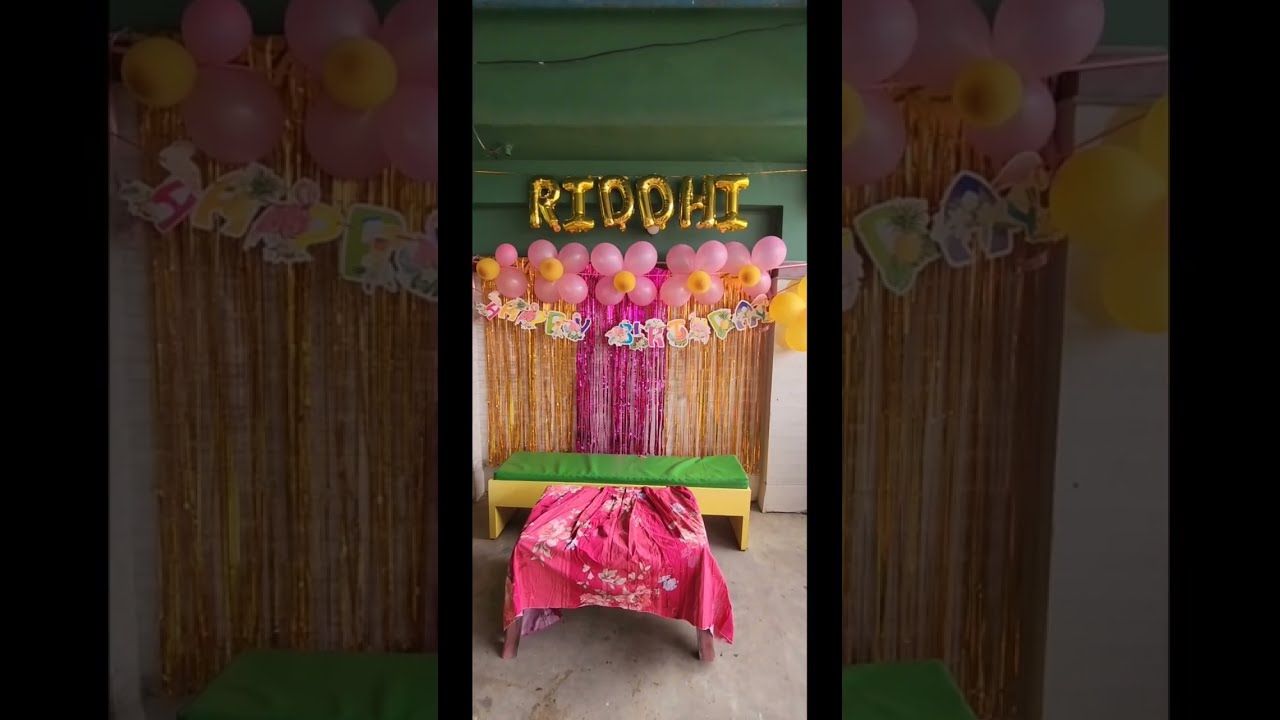In the image, a detailed birthday setting is depicted with a picture-in-picture composition. The central focus is a room interior adorned for a celebration. The ceiling and the top of the walls are a darker, green color, contributing to the festive atmosphere. Front and center, gold balloons spell out "RIDDHI", with each letter individually formed. Beneath this, a charming array of balloon flowers, featuring pink petals and a yellow center, creates a vibrant row—though the flower on the far left appears slightly deflated. Streamer-like tinsel in gold and pink drapes gracefully down the length of the wall.

Below this colorful display, a green and yellow bench sits prominently in front of a small table which is dressed with a pink tablecloth adorned with white flowers. The floor beneath appears to be a light sand or concrete color. Adding to the tropical theme are cardboard cutouts of birds and a bamboo backdrop, painted purple in the middle. A "Happy Birthday" banner is also strung across the patterned bamboo. The overall scene is a cheerful mix of textures and hues, perfectly set for a joyful celebration.